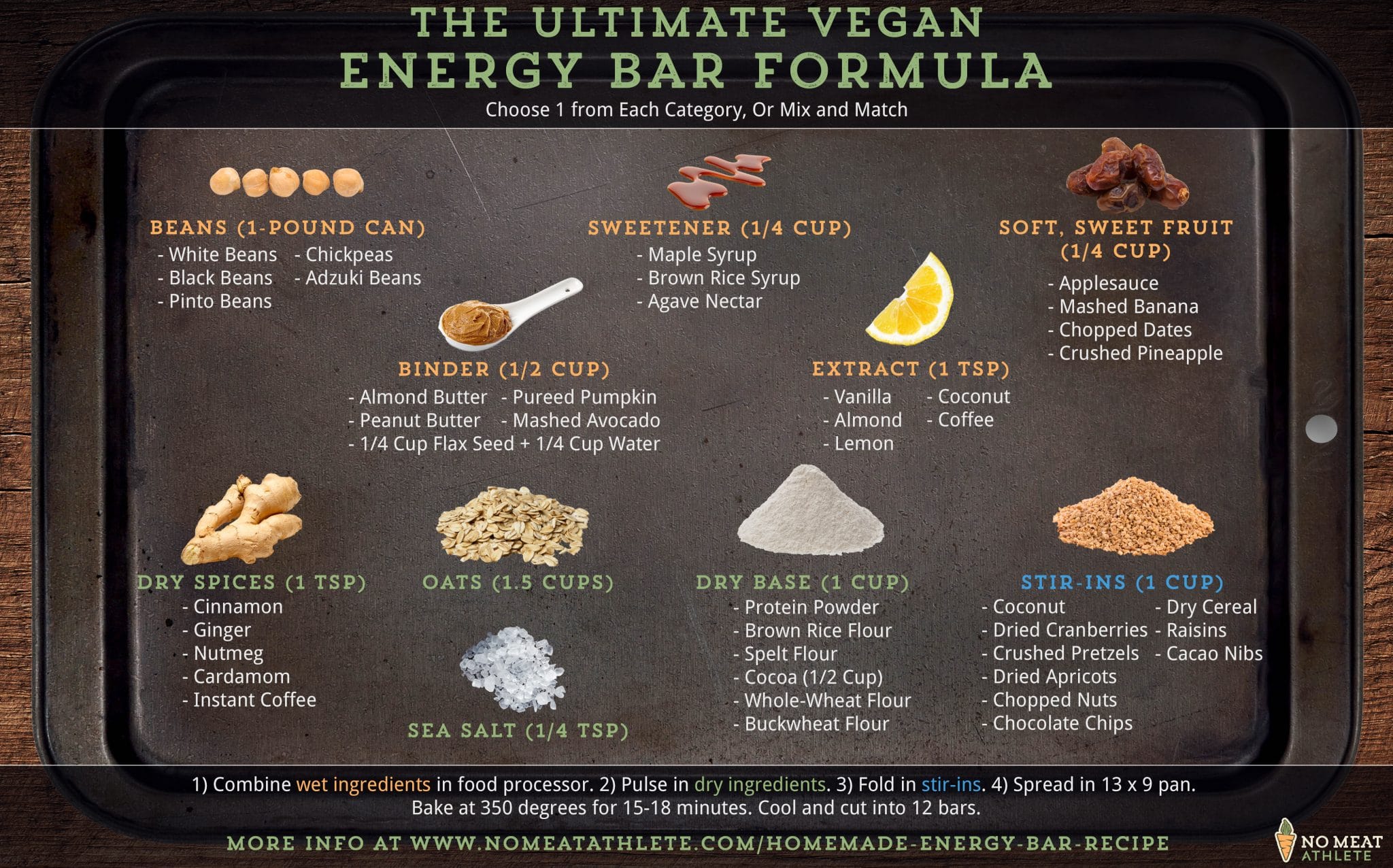This informative infographic, set against a black landscape background, details "The Ultimate Vegan Energy Bar Formula" in green text at the top. Below that, in white text, it instructs to "choose one from each category or mix and match." Centered on a dark silver baking sheet atop a dark brown wooden table, photographs of various food items are organized into categories: beans, sweeteners, soft sweet fruits, binders, extracts, dry spices, oats, dry bases, stir-ins, and sea salt. Each category, highlighted in orange, green, or blue text, includes detailed bullet points with specific examples like white beans, black beans, and pinto beans under the beans category. In the lower right corner, there's a colorful logo in white, orange, and yellow, while the bottom contains further instructions in white text. To discover more recipes, a website link directs to nomeatathlete.com/homemade_energy_bar_recipe.